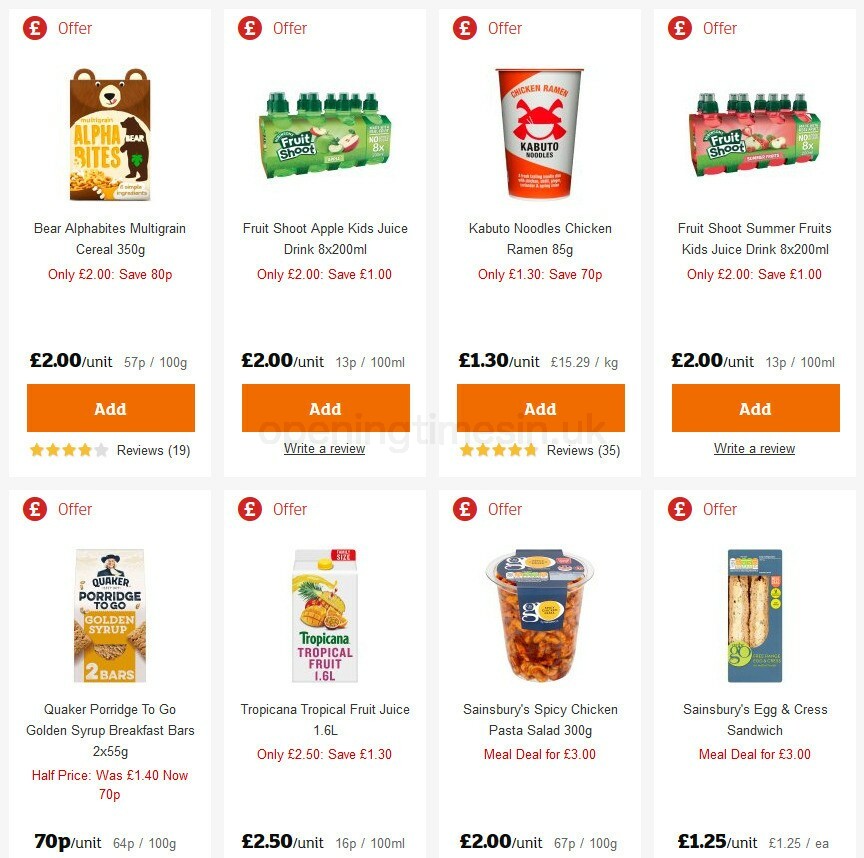A screenshot from a food or grocery shopping website displaying a selection of products neatly arranged in two rows, with four items per row, against a white background. Prominent orange "Add to Cart" buttons with white lettering are visible under each item.

**First Row:**
1. **Bear Alpha Bites Multi-Grain Cereal**  
   Price: $2 per unit
2. **Fruit Shoot Apple Kids Juice Drink**  
   Price: $2 per unit
3. **Kabuto Noodles Chicken Ramen, 85 grams**  
   Price: $1.30 per unit
4. **Fruit Shoot Summer Fruits Kids Juice Drink**  
   Price: $2 per unit

**Second Row:**
1. **Quaker Porridge to Go Golden Syrup Breakfast Bars**  
   Discounted Price: 70p (originally $1.40)
2. **Tropicana Tropical Fruit Juice**  
   Price: $2.50 per unit
3. **Sainsbury's Spicy Chicken Pasta Salad, 300 grams**  
   Meal Deal: £3, Regular Price: $2 per unit
4. **Sainsbury's Egg and Crust Sandwich**  
   Meal Deal: £3, Regular Price: $1.25 per unit

This organized layout provides a quick and clear snapshot of a variety of food items available for purchase, complete with prices and brief descriptions.